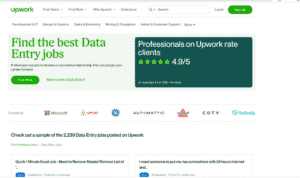The image shows a webpage from Upwork, though the resolution is quite low, making most elements difficult to discern. At the top are four white buttons featuring black text, followed by a search bar and a green button positioned on the right. Below this section are six black-on-white navigation tabs, although their text is unreadable. The page prominently displays the phrase "Find the best data entry jobs" in green text, accompanied by an illegible black subtitle. Another green button is present here. To the right, text reads "Professional professionals on Upwork great clients 4.9/5" with accompanying green stars. This content is set against a dark hunter green background with white font. Further down the page, additional buttons are partially visible, with one likely representing Microsoft's logo and another labeled as "Cody." The rest of the buttons and content are unclear, displaying a mixture of green, white, black, blue, and red colors.